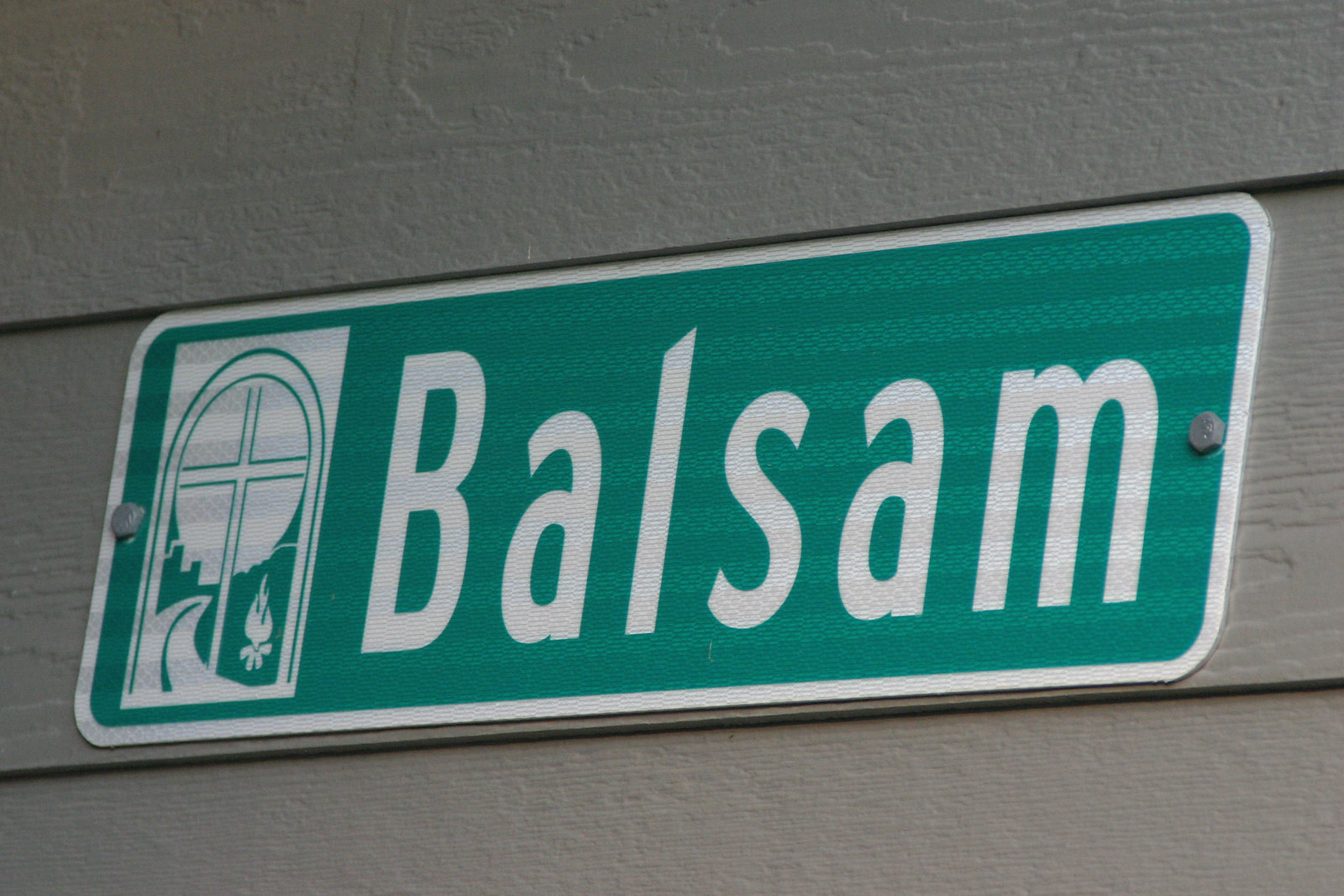Three distressed white wooden planks form the backdrop of this image, their ingrained texture suggesting they might be made of a resilient resin. In the foreground, a retro-style green sign is affixed to the planks with two silver rivets. The sign is rectangular with rounded corners and has a classic white border, commonly found on street or informational signs. 

The green sign, printed with reflective material, features two variegated stripes and a protective coating that give it a weathered, yet durable appearance. On the left side of the sign, a detailed, mixed logo is depicted: an arched window containing a white cross, a white sun, trees, a curved roadway, and a small campfire with logs at the base. This imagery suggests that the location could be either a church or a campground, possibly both.

To the right of the emblem, in bold white text, the word "Balsam" is prominently displayed. The overall combination of design elements and the name indicates a serene, multifaceted location likely named Balsam.